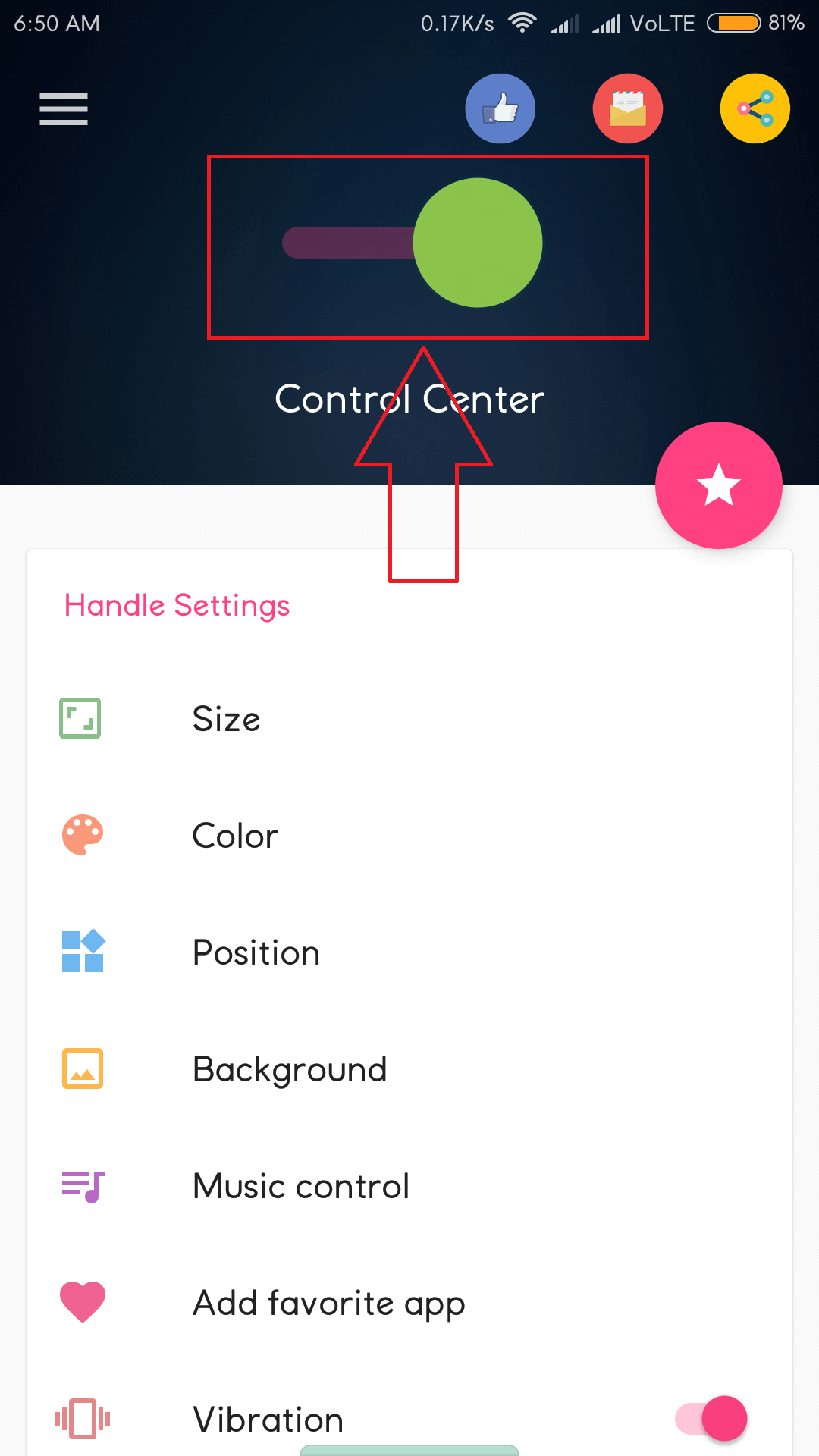Screenshot of smartphone at 6:50 AM with 81% battery and a dark grey background. Top left features a "hamper" button. Visible icons include: a blue circle with a thumbs-up, a red circle with an envelope and letter, and an orange circle with a share icon. Below, there's a toggle bar in green, switched to the right, encased in a red rectangular box with an upward-pointing red arrow at the bottom. Text below the toggle bar reads "Control Center". Further down, a pink circle with a white star and text "Handle Settings" in pink. Listed options include: Size, Color, Position, Background, Music Control, Add Favorite App, and Vibration. A pink toggle bar to the right of "Vibration" is switched to the right.